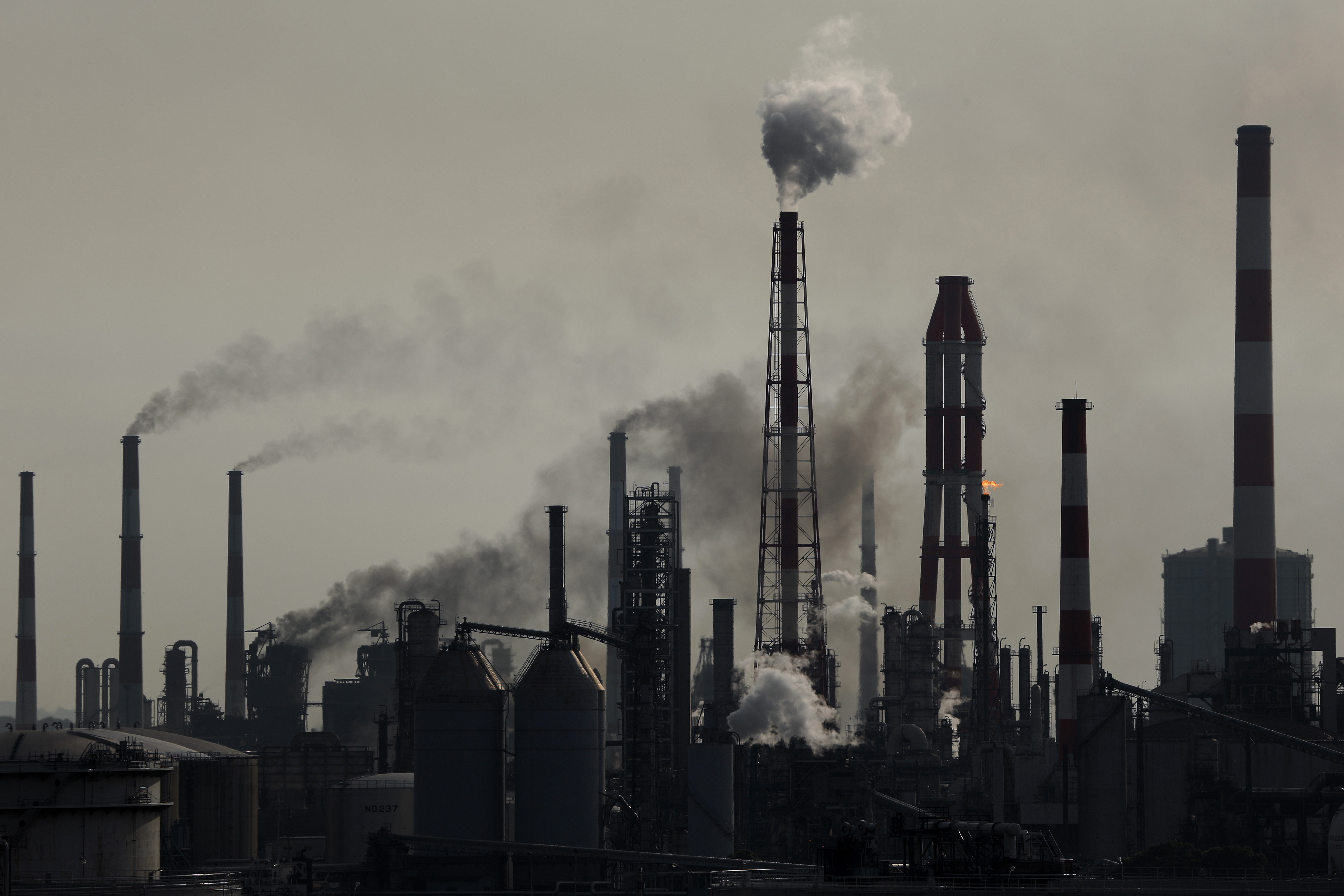The image depicts a distant view of an oil refinery shrouded in a high-contrast, almost monochrome aesthetic, likely taken through a filter that enhances the starkness of the scene. The sky is an ominous gray, devoid of discernible clouds, contributing to the industrial, almost dystopian atmosphere. The refinery itself is silhouetted against this dark backdrop, with an array of thin chimneys prominently featured. Smoke billows from chimneys primarily on the left and center of the image, adding to the smoky, murky sky. On the right-hand side, a chimney striped with black or white and red bars stands out, lacking the smoke that emanates from its counterparts. A touch of fire flickers near the center-right, hinting at the refinery's continuous operations. Several smokestacks are isolated, while others are enveloped by trellis work, suggesting access structures for maintenance purposes. The absence of people and identifying text further accentuates the bleak, industrial landscape, reminiscent of scenes from the industrial revolution, but firmly set in the modern day.